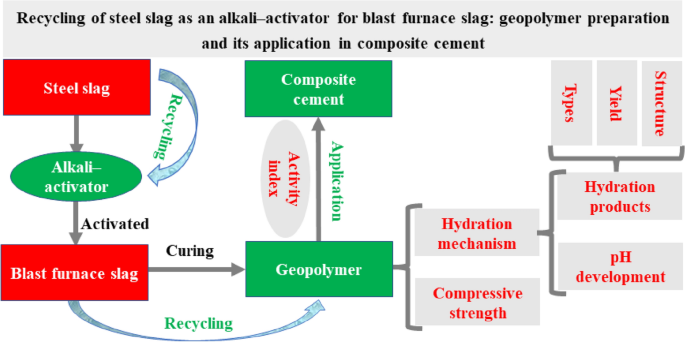The image presents a detailed flowchart of chemical manufacturing processes focused on the recycling of steel slag as an alkali activator for blast furnace slag. At the top, the chart is labeled: "Recycling of Steel Slag as an Alkali Activator for Blast Furnace Slag: Geopolymer Preparation and Its Application in Composite Cement." The flowchart illustrates the journey of steel slag being processed into an alkali activator, depicted by a red square leading to a green oval labeled "alkali activator," and then to a red rectangle labeled "blast furnace slag" with arrows indicating the stages of recycling and curing. The process continues with an arrow pointing from "blast furnace slag" to a green oval labeled "geopolymer," and further to a rectangle indicating "composite cement," with notes on its application and activity index. On the right side of the diagram, smaller boxes detail additional aspects of the process, such as "structure," "yield," "types," "hydration products," "pH development," "hydration mechanism," and "compressive strength," forming a comprehensive visual guide to the recycling and transformation of steel slag in the context of cement production.